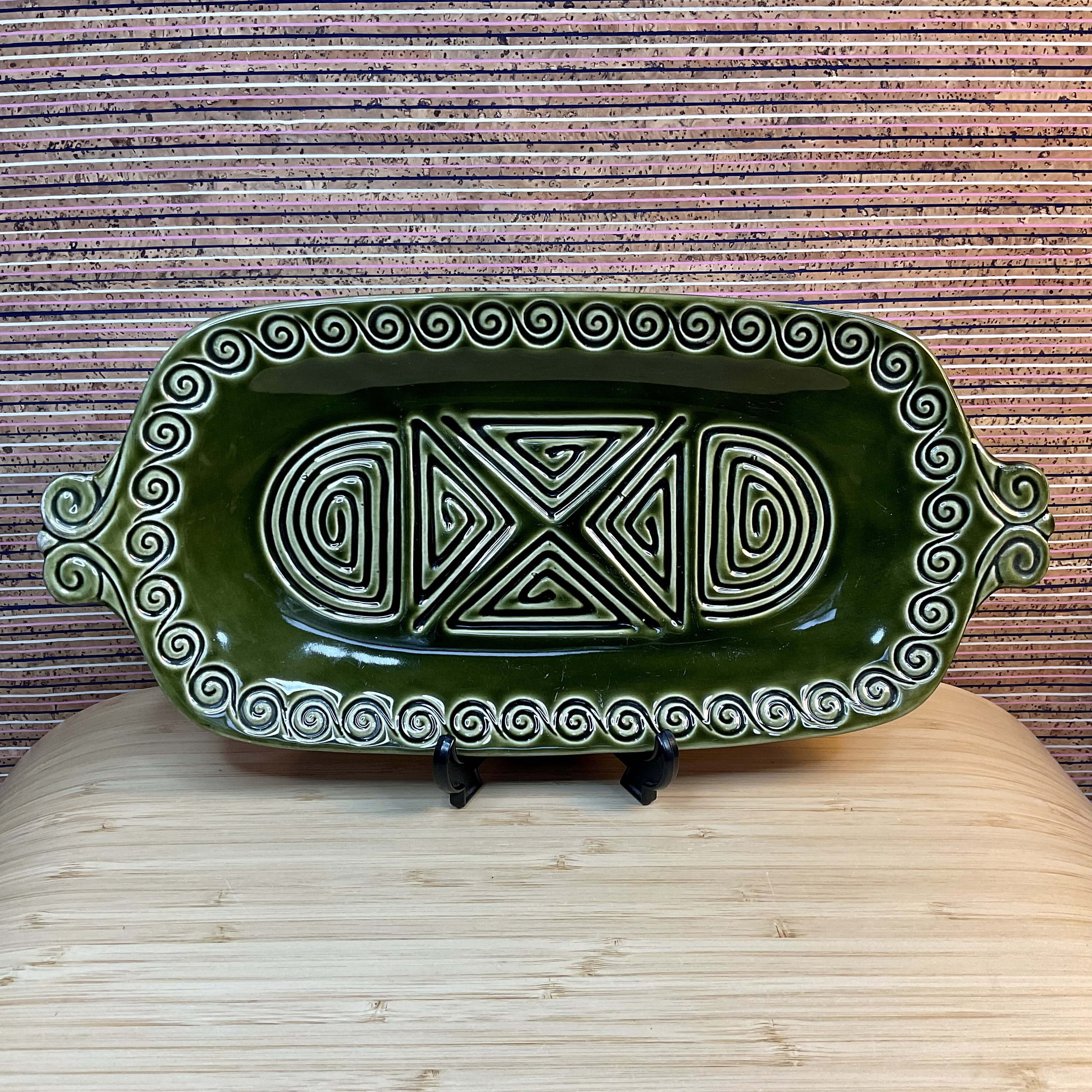The image displays a photograph of a decorative serving dish, positioned on a light, shiny wooden surface with visible grain. The dish, oblong in shape and reminiscent of a lasagna pan, is propped up on a black easel stand. The background features a pink, white, and black striped pattern, possibly fabric or wallpaper. The dish itself is dark green with intricate white swirly designs, resembling rolling waves, adorning its edges. It also has two protruding handles, each embellished with a similar patterned design but in green. In the center of the dish, a square is formed by four triangles, each with lines running through them, arranged in an X pattern. Surrounding this central motif are half-circle designs that spiral outwards, like tiny cinnamon rolls.